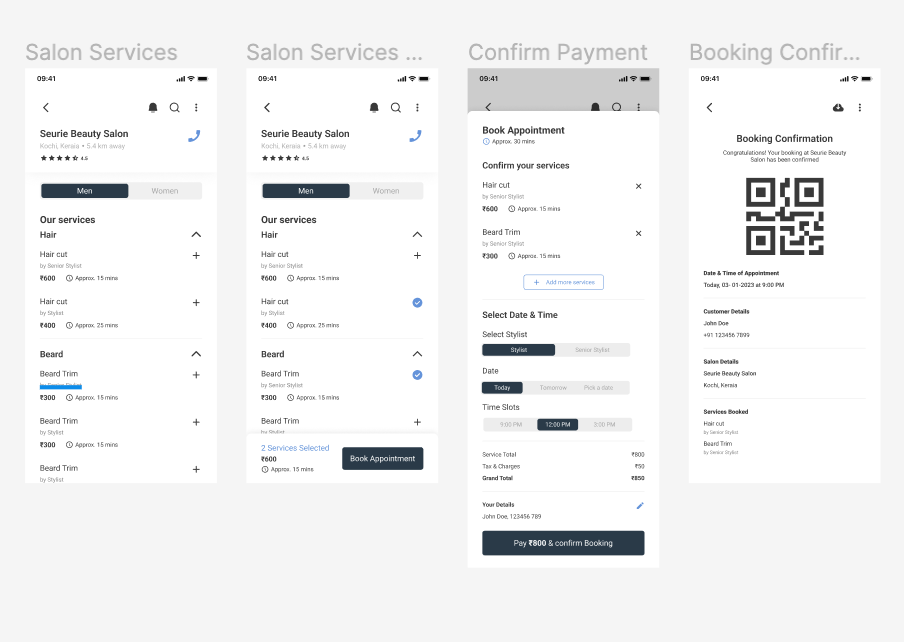The image features a collage of four smartphone screens, meticulously arranged side-by-side in a 1-2-1 grid formation. The far-left screen displays the heading "Salon Services" in gray, showcasing a page for "Siri Beauty Salon," specifically highlighting services for men rather than women. This screen details some of the salon's offerings, such as haircuts, which take approximately 15 minutes and are priced at 600 and 400 units of an unspecified currency. Additionally, it mentions beard trims, although part of this section is obscured by a blue marker, suggesting an adjustment or correction made by the user.

The two middle screens display similar content. The first one reiterates "Salon Services" for "Siri Beauty Salon," allowing users to book appointments directly. Beside it, the second screen shows a confirmation of a payment and a booking confirmation, indicating that a service has been successfully reserved and paid for.

Overall, the image appears to document a detailed overview and management of salon services and appointments, possibly for record-keeping or administrative purposes.